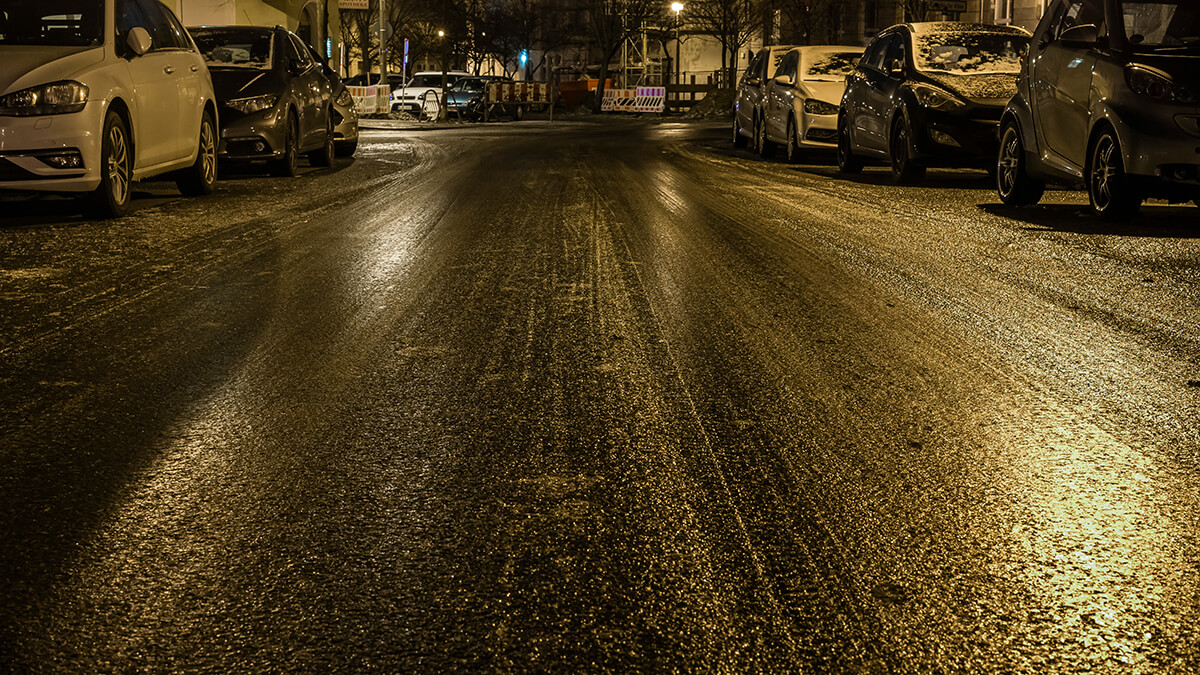The image depicts a nighttime scene of a wet, possibly icy city street, reflecting the yellow glow of overhead streetlights. The asphalt, glistening with ice crystals, adds to the overall yellow cast of the scene. The street, likely a one-way road as the cars are all uniformly parked facing the same direction on both sides, extends toward an intersection. The vehicles, including a mix of white, black, gray, and a small electric car, are lightly dusted with snow. In the distance, a building with a sign and additional parked cars on a diagonal street can be seen. Near the end of the street, there is a parking lot with a white SUV. The overall atmosphere is quiet, highlighted by the stillness of the parked cars and the glistening wet surface of the road under the street lamps.